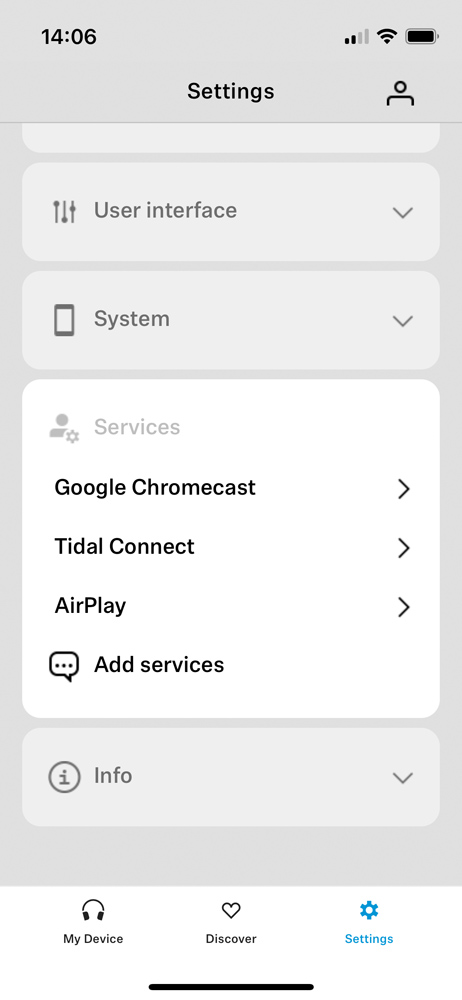A user posted a screenshot of their phone's settings menu, evident from the visible Wi-Fi and cellular signal bars in the top right corner, along with the battery life indicator. The phone is likely an Android device, inferred from the presence of Google Chromecast under the services options. The screenshot highlights the services submenu within the settings, showing available choices such as "Connect," "Airplay," and "Add Services." The detailed view includes various sub-options, expanding the services menu while other sections remain minimized to optimize screen space. Notably, at the bottom of the screen, a light blue-highlighted option titled "Discover a Setting" stands out, flanked by two grayed-out alternatives.